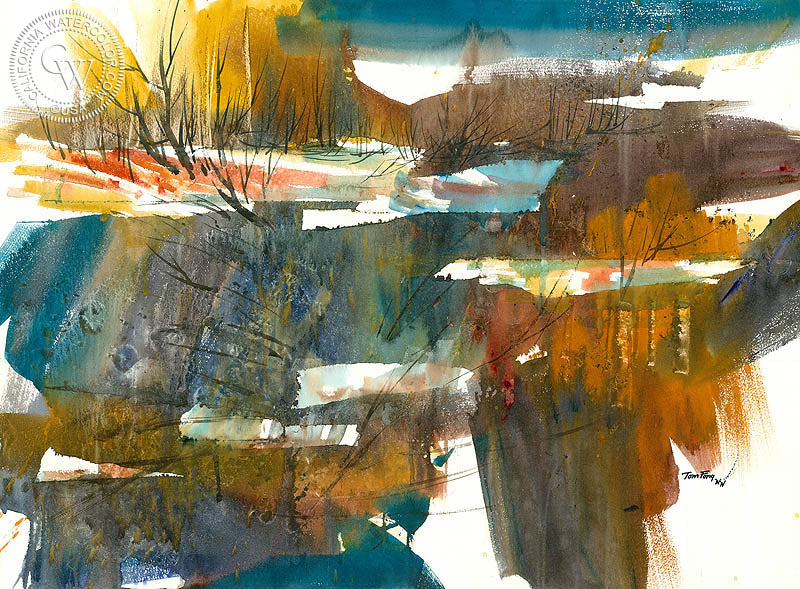This abstract watercolor painting features a dynamic composition of earthy and vibrant tones against a white backdrop. Dominated by rusty oranges, mustard yellows, deep turquoise with hints of green, and various shades of brown, the artwork evokes a sense of autumnal landscapes and natural elements. The upper left corner is marked with a circular seal that reads "California Watercolor dot com" encircling the initials "CW" along with "copyright USA."

Prominent are the brush strokes and shapes suggestive of bare trees or twigs, densely layered to create an impression of sparse, tall grasses. These elements are scattered with an interplay of turquoise and earthy colors, adding a sense of movement and depth, as if depicting changing seasons or land and water intermingling. The overall effect is a harmonious yet chaotic mix, where the shapes and colors blend to form a piece that captures the fluidity and essence of nature in an abstract manner.